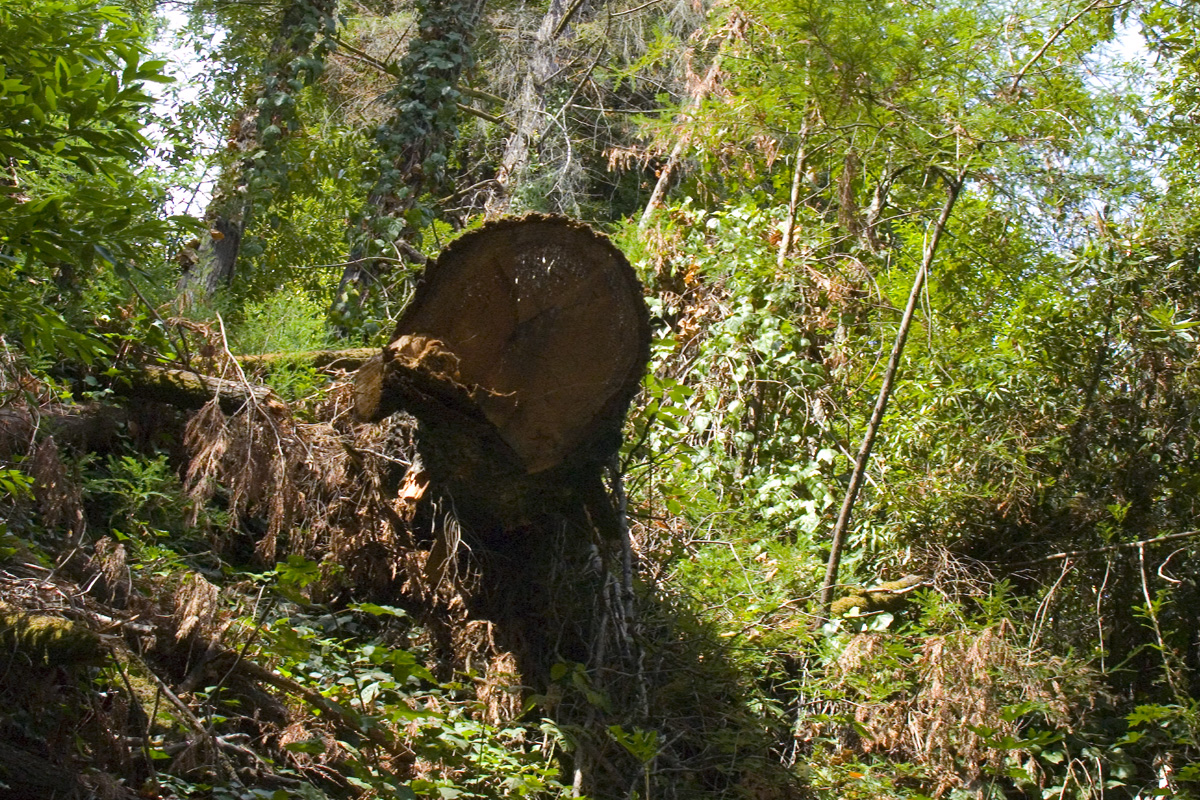This vibrant and detailed forest scene centers around a large, cut tree stump, its cross-section revealing the intricate rings of growth. Surrounding the stump are numerous dead branches, emphasizing a sense of natural decay. Encircling this focal point is a rich, dense forest teeming with tall, green trees, some dotted with vines, and a variety of other vegetation, including bushes, ferns, and grass. A mix of living and dead trees adds variation, with splashes of brown interspersed among the green foliage. The bright and sunny setting is further highlighted by patches of blue and white sky visible in the upper corners, indicating a clear, well-lit day. The lower half of the image features additional fallen branches and low-lying plants, contributing to the overall lush and vibrant yet rugged appearance of this forest clearing.